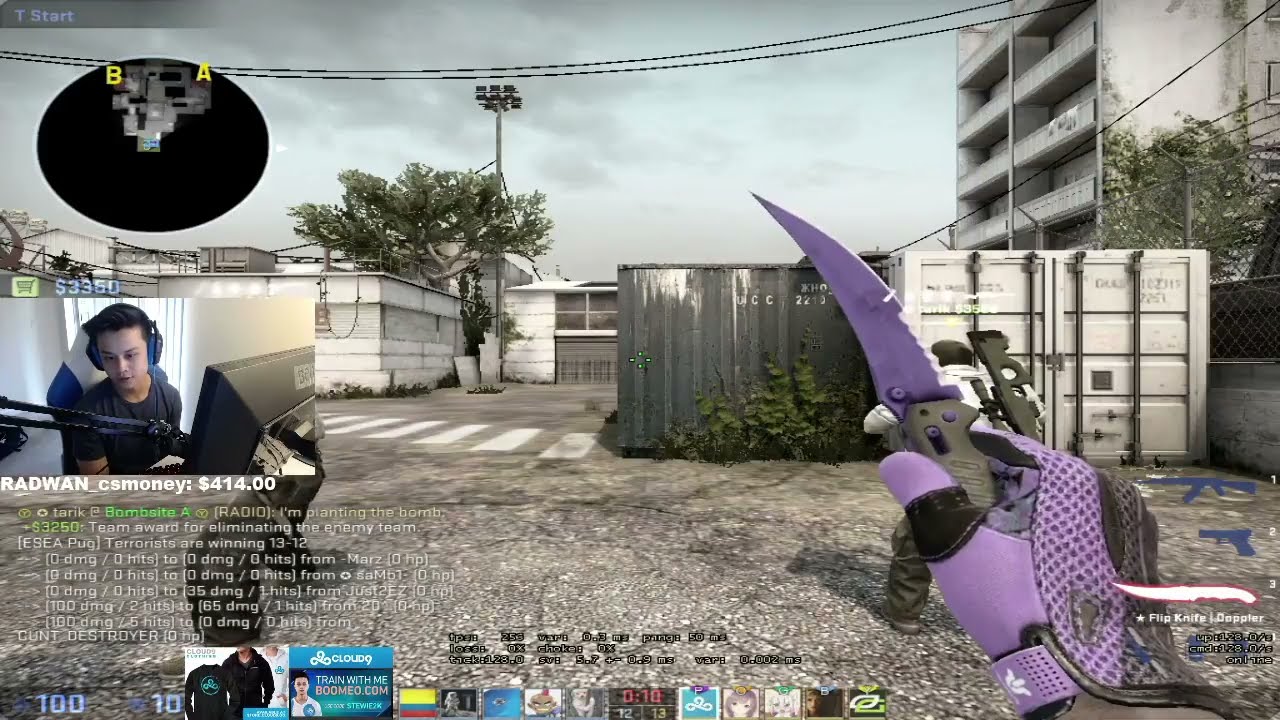In this detailed image from a video game, the primary scene features an urban environment with buildings and shipping containers. The ground is a rough, gravelly pavement, and a white-striped crosswalk runs through the center. On the right side, there's a storage building and a large white apartment building, standing four stories high. Telephone wires crisscross the hazy white sky, supported by a pole with speakers or lights.

A character dressed in a dark white jacket, black pants, and a baseball-type hat is seen moving away from the viewer on a purple motorcycle, with one foot touching the ground. Another character's hand, wearing a purple leather glove with black knuckles, holds a knife with a dark gray base and a purple blade visible on the right side of the screen.

On the left side of the image, there's an inset showing a young man with dark hair and headphones, likely the streamer playing the game. He is sitting in a gaming racing-style chair, facing a computer monitor with a microphone in front of him. This inset is filled with various text, numbers, and images, including a dollar figure of $414 and a mini-map above the streamer's head. There are letters "B" and "A" in gold within a black oval at the top left corner of the image. The intricate layout and details suggest a dynamic first-person shooter game being live-streamed.